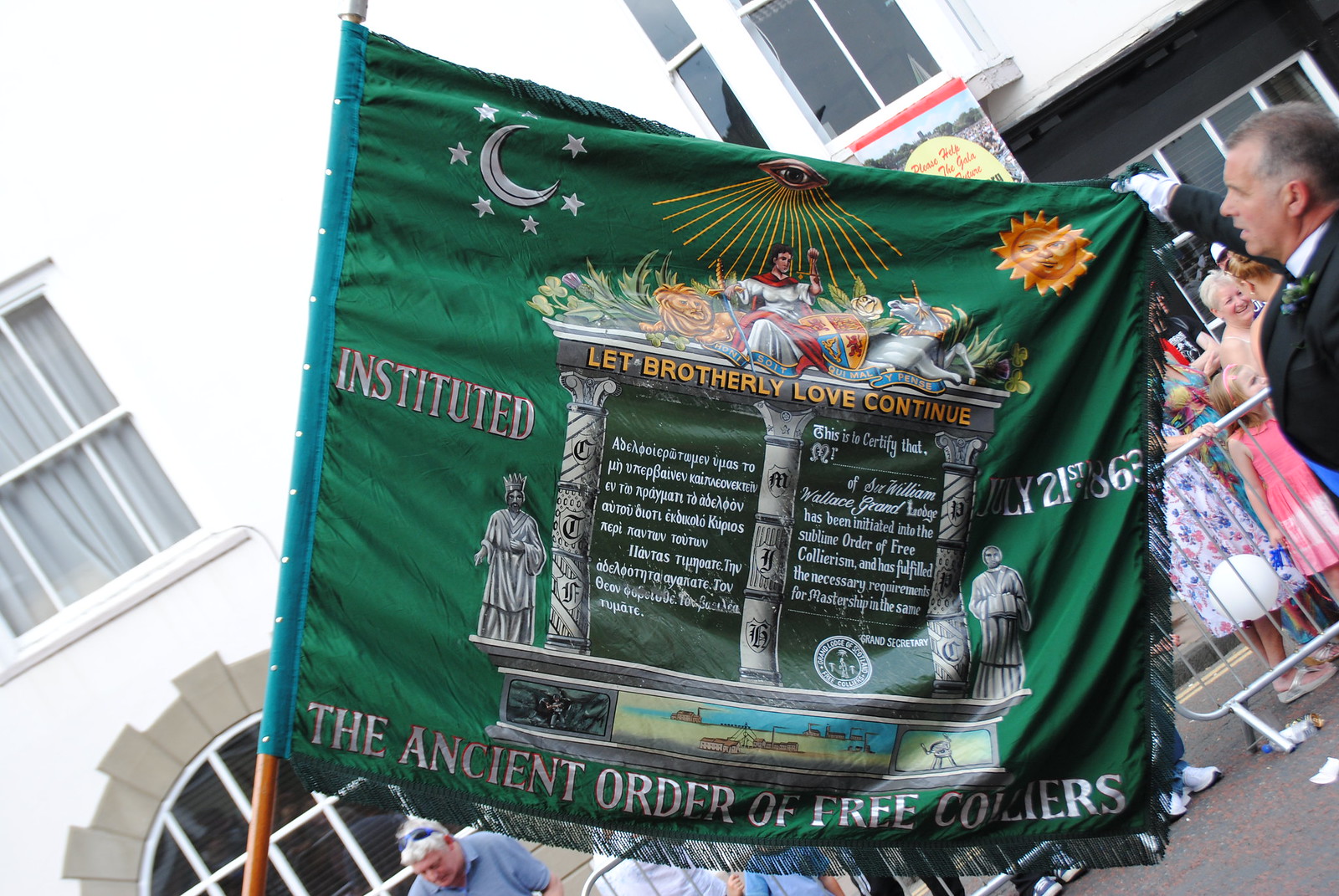In the image, a daytime outdoor scene depicts a dark green flag mounted on a wooden pole, being held at the corner by a man in a black suit with white gloves. The flag features intricate designs and text, including three gray stone columns supporting an overhead structure. At the center top of the flag, an illustrated eye with yellow rays emanates from it, flanked by a silver crescent moon with stars on the left and an orange sun with a face on the right. Below this celestial imagery, a man in a white robe and red scarf sits on a stone building beside a colorful shield adorned with a golden lion on the left and a white unicorn on the right, surrounded by green leaves. On the flag’s lower portion, silver or gray inscriptions include "Let Brotherly Love Continue" and other text in a foreign language. The date "July 21st, 1863" and phrases such as "Instituted," "The Ancient Order of Free Collierism," and a certification statement about the initiation into the order are also visible. The flag is fringed on three sides and folds obscure some text. In the background, a white building and a temporary metal barricade hold back spectators, suggesting the setting might be a parade.